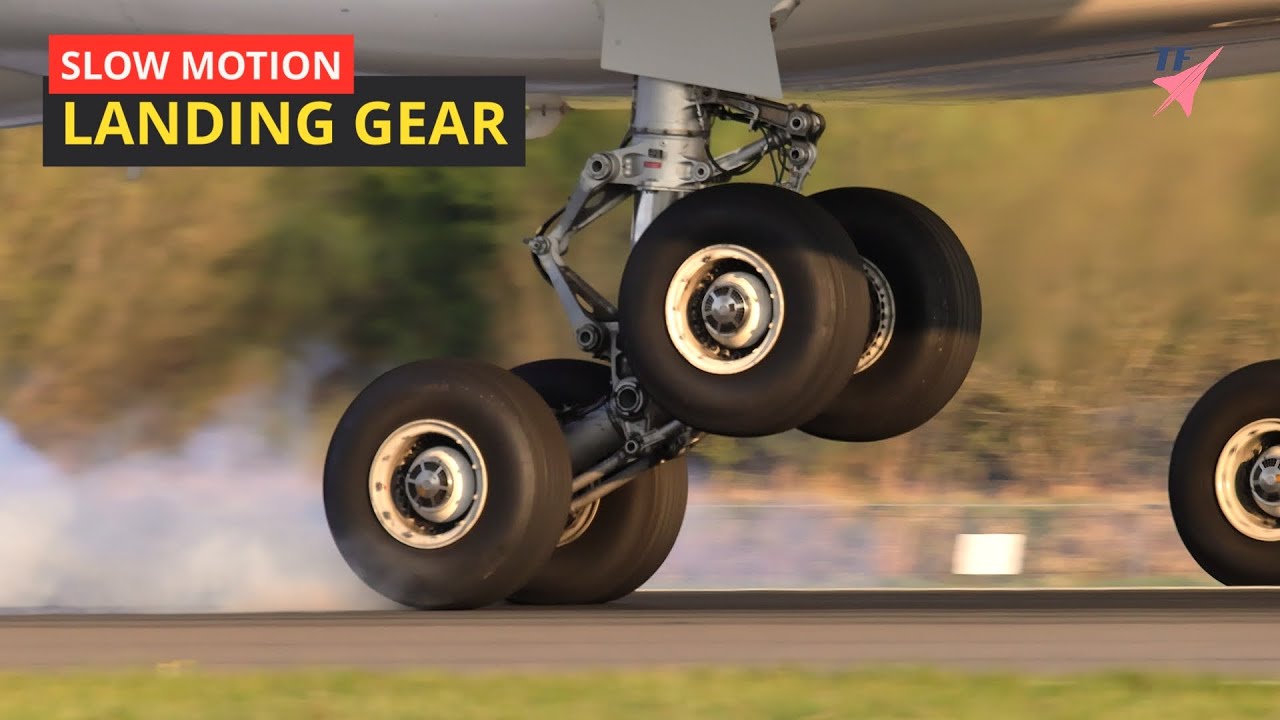This detailed photograph, clearly taken outdoors, captures the dramatic close-up of an airplane's landing gear in action. Dominating the upper left corner, the text "Slow Motion" appears in white uppercase letters within a red box, while just below, the words "Landing Gear" are displayed in a black box with yellow uppercase lettering. Both captions combine to read "Slow Motion Landing Gear." The image reveals the rear two tires of the landing gear making contact with the ground, producing significant white smoke as they skid along the tarmac. The two front wheels, still hovering just above the ground, suggest the dynamic moment of descent and landing. The photograph also includes a streak of light brown tarmac and a thin strip of grass at the bottom, with the blurred background indicating the plane's motion. Additionally, the upper right corner features a blue logo with "TF" and a small airplane symbol. The hydraulics and a portion of the aircraft’s underbelly are visible, enhancing the detailed portrayal of this crucial moment in aviation.